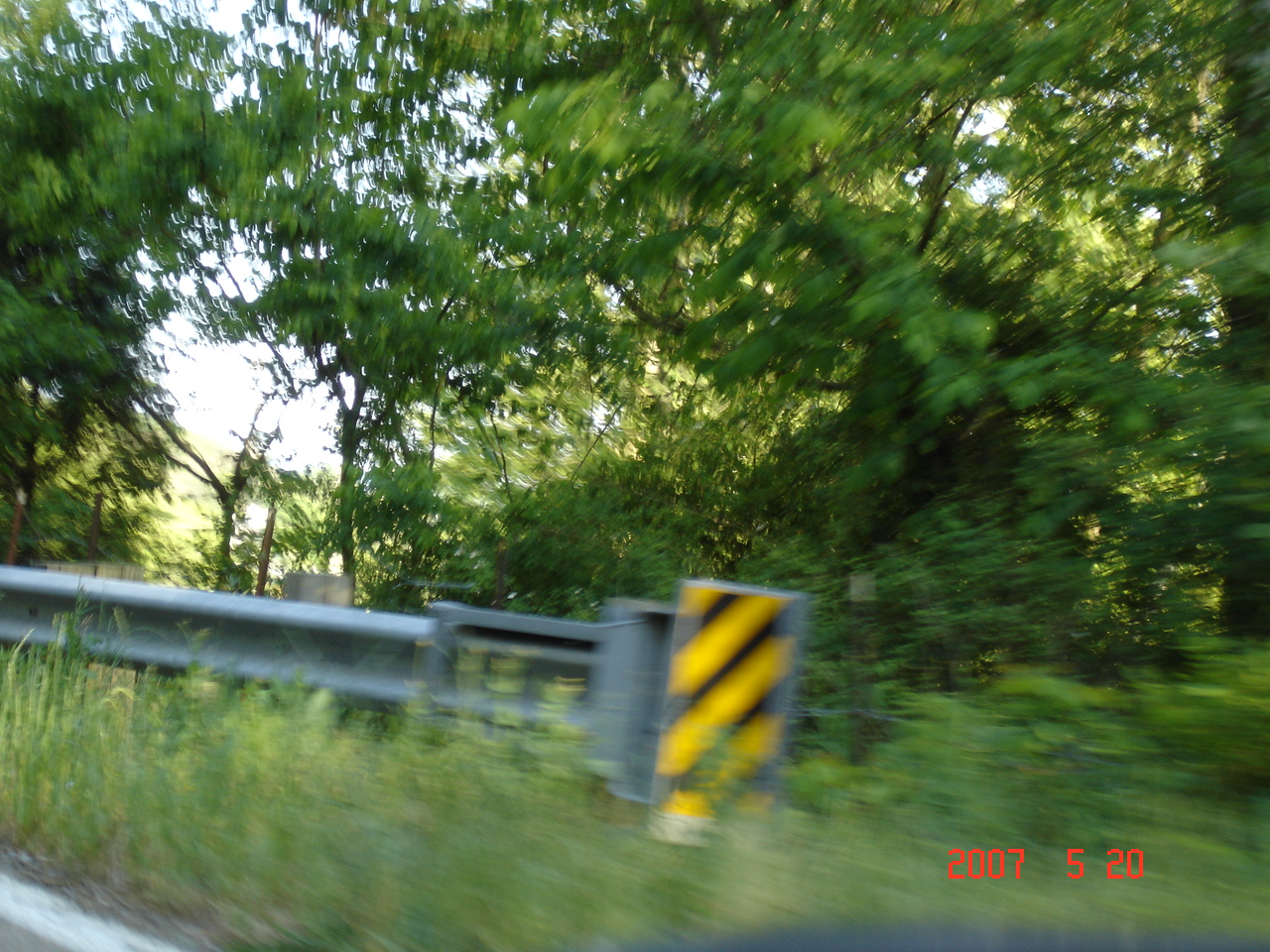Captured on May 20, 2007, this photograph, snapped from a moving car, vividly illustrates the fleeting scenery outside. The motion of the vehicle is evidenced by the blurred images of the landscape, creating a dynamic sense of movement. A distinctive yellow and black bumper is prominently positioned against a gray metal guardrail. Below the guardrail, a white curb sharply delineates the road from the surrounding terrain. The sky above is a muted gray, casting a subdued light over the scene. The view is dominated by an abundance of verdant trees and high, overgrown grasses that reach up to the base of the guardrail. Below, wild weeds thrive along the roadside, adding to the sense of untamed nature. Beyond the dense greenery, the landscape fades into obscurity, offering no further details of what lies ahead.